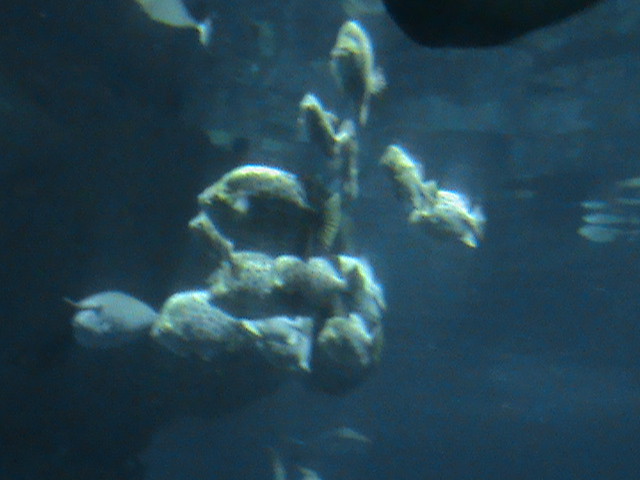This underwater photograph, rendered in dark blue hues, is quite blurry, making it challenging to discern specific details with clarity. The image appears to depict an underwater structure, possibly a piece of coral or a rock, with a greenish tint at the bottom. There are approximately half a dozen silvery gray fish with spots swimming around the focal structure, along with a smaller school of fish gathered towards the center-right edge of the frame. The underwater scene is somewhat obscured by the poor focus, leaving the exact nature of the sea life somewhat ambiguous.